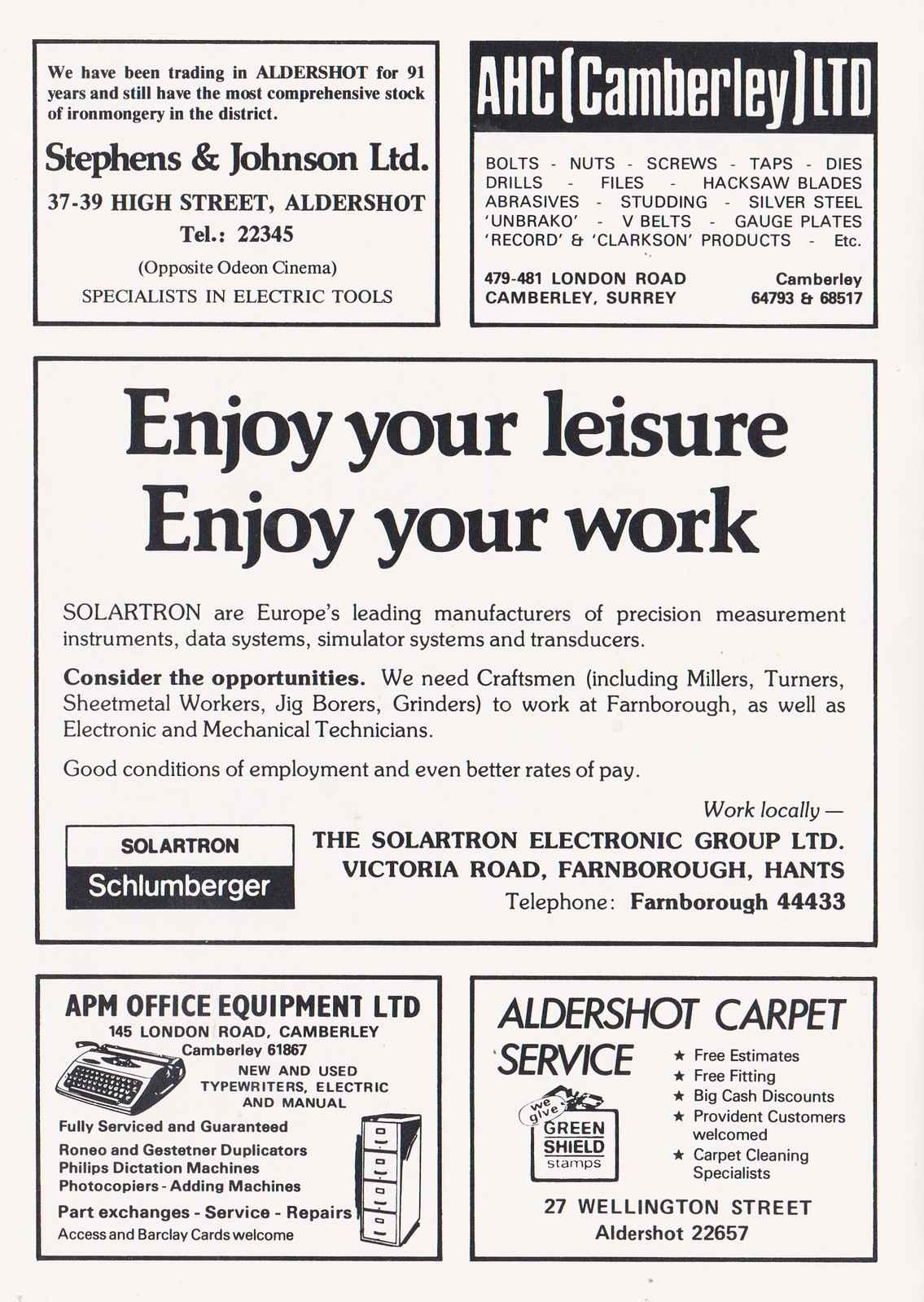This is an old page from a magazine, specifically an official program booklet from a soccer game, filled with five distinct advertisements. At the top left, the ad for Stevens & Johnson Ltd. states, “We have been trading in Aldershot for 91 years and still have the most comprehensive stock of ironmongery in the district.” Next to it, on the top right, is an ad for AHC, Camberley Ltd., listing various products such as bolts, nuts, screws, taps, dies, drills, files, hacksaw blades, abrasives, studding, silver steel, v-belts, gauge plates, and more, indicating its address on London Road in England. Dominating the center of the page is a larger advertisement that spans about two-thirds of the space, proclaiming, “Enjoy your leisure, enjoy your work,” and promoting Solartron, Europe's leading manufacturer of precision measurement instruments, data systems, simulator systems, and transducers. At the bottom left is an advertisement for APM Office Equipment Ltd., offering a full service guarantee. Finally, on the bottom right is the advertisement for Aldershot Carpet Services, featuring free estimates, free fitting, big cash discounts, and services for Provident customers, located at 27 Wellington Street.